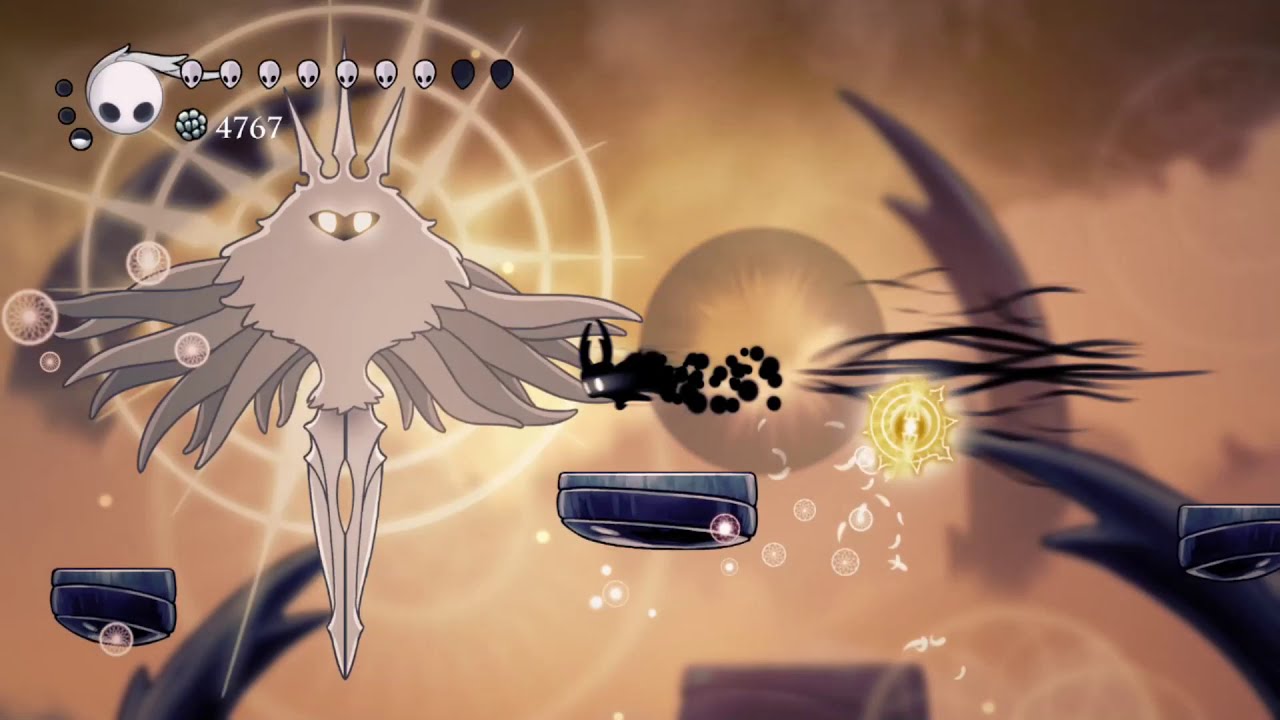In this game-themed cartoon image, we see a detailed scene with a predominantly gold and yellow background. Dominating the center is a large, darker grayish planet or moon. To the left, there’s a prominent mythical figure resembling a lady but with fantastical features: multiple wings and legs, two glowing eyes, three spikes atop its head, and tentacle-like appendages. This figure has a narrow waist adorned with fringes and long pointed legs. Above this creature is the number 4767, indicating it's part of the game interface.

On the upper left of the image, there are ten skull icons, seven of which are white with dark eyes and three black ones, possibly representing game lives or progress. Next to these is a larger skull with a white background and two dark eyes. Along the left side, there’s an array of zodiac-like, sun symbols and circular designs which appear brighter than their surroundings.

Interspersed throughout the scene are purply-bluish objects, including sorcery-like shapes and discs resembling off-center rings, contributing to the mystical atmosphere. Additional circular and horn-like patterns behind the central figure add to the intricate and fantastical nature of this game-themed artwork.